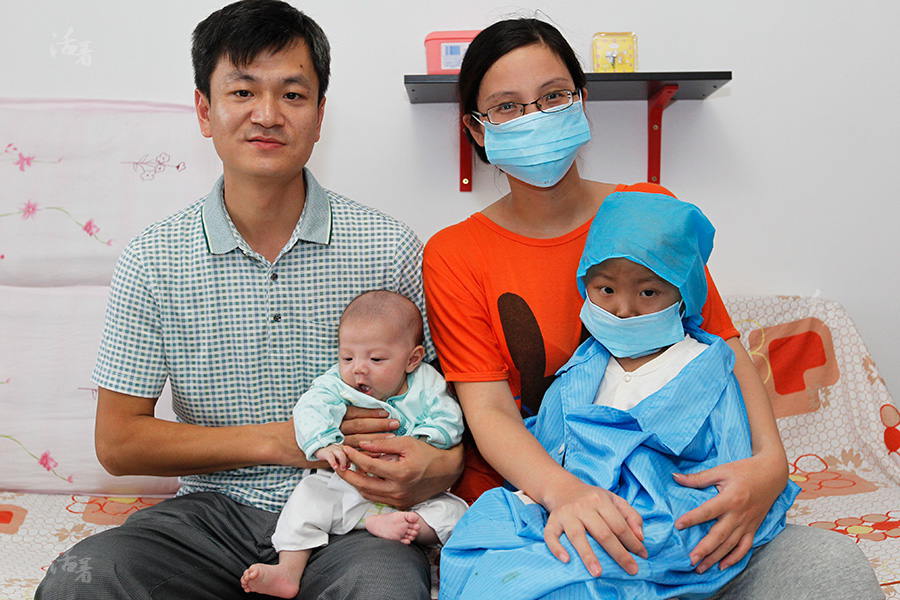This image depicts an Asian family of four sitting in a room with white walls adorned with pinkish decorations. The father, positioned on the left, cradles a very young baby in a light blue onesie, while the mother, on the right, holds a small child, possibly around four or five years old, who is dressed in blue surgical clothing, including a gown and cap, and wears a blue surgical face mask. The mother is also wearing a blue surgical face mask and is dressed in an orange t-shirt with black accents. Both parents, who have black hair and the mother wears glasses, appear to be smiling affectionately, with the mother’s smile evident through her eyes. They are seated on a couch covered with a decorated coverlet. Behind them is a small bookshelf with a black panel, red brackets, and a clock in a yellow box along with a pink box, which adds more detail to the room’s ambiance, possibly indicating a hospital or residential setting. The intimate setup and the protective gear worn by the mother and child suggest a careful and caring environment, likely influenced by health considerations surrounding the child.